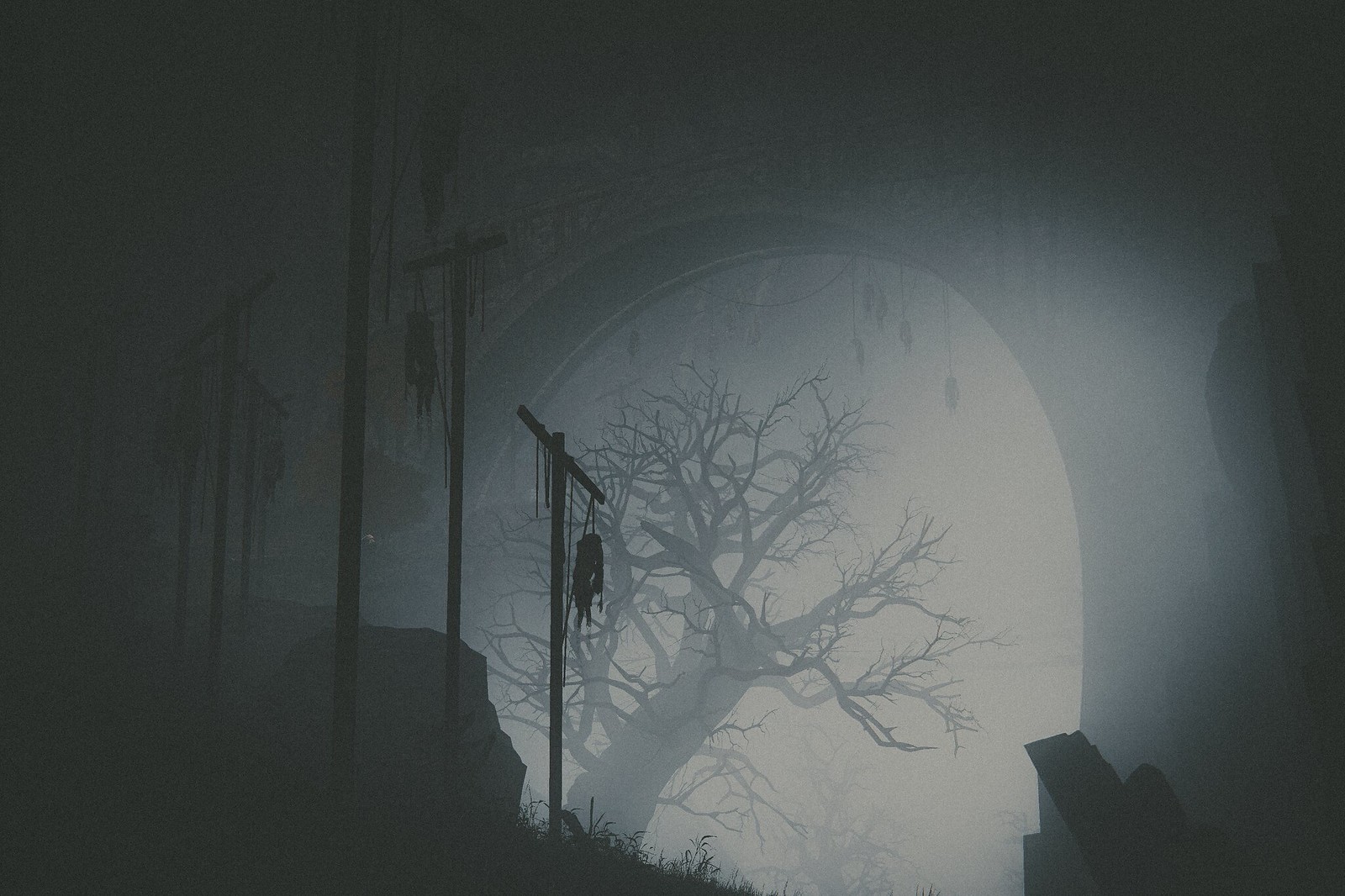The image captures an intense, gothic ambiance with its dark and moody presentation. Dominating the foreground is a large, shadowy archway that looms imposingly, casting a deep shadow and creating a stark, dramatic frame for the scene. Through the archway, a haunting landscape unfolds, shrouded in mist and exuding an eerie stillness. Silhouetted against the foggy backdrop are gnarled, leafless trees, their twisted branches adding to the sense of desolation and mystery. Enhancing the macabre atmosphere, there are unsettling figures hanging from the archway and nearby structures, possibly indicating a grim fictional setting or horror-themed decoration. The color palette is subdued, composed of various shades of gray and black, further reinforcing the chilling, spectral mood of the scene.